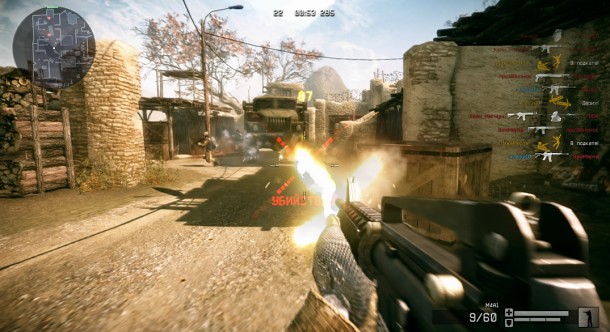The image illustrates an intense moment from a first-person shooter (FPS) video game. In the foreground, a gloved hand extends from a sleeved arm, gripping the front section of a sleek, black automatic rifle. The muzzle of the gun is ablaze, discharging bullets toward a distant red X marker that is accompanied by cryptic numbers and letters. The scene appears to be set in an outdoors area featuring a dirt road. Further back, there is an armored vehicle and a soldier, hinting at an active combat scenario.

The environment is detailed with stone walls in a beige hue and a wooden crate to the right. To the left, there's a small platform area with chopped wood. A single tree and a power line with a street light add realism to the background, while a towering mountain looms under a blue sky streaked with white clouds. The image also displays a user interface (UI): a mini-map on the left side of the screen and weapons information on the right, aiding the player's navigation and strategy.